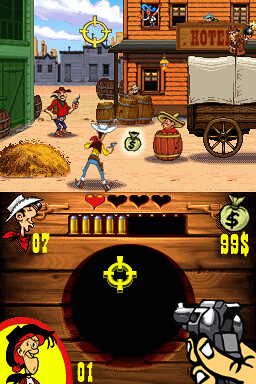This image comprises two stacked panels, each depicting a scene from a cowboy-themed cartoon set in an old Western town. 

In the top panel, a tense standoff unfolds: a cowboy with a white hat and holsters, gun drawn and aimed, stands opposite a man emerging from a barrel wearing a sombrero. Between them lies a yellow bag marked with a money symbol. A third cowboy, also armed, is visible in the left background, enhancing the suspense of the confrontation. The backdrop features a rustic building with a prominent "Hotel" sign, cementing the Old West atmosphere.

The bottom panel focuses on close-up facial expressions of two cowboys, one on the left and the other on the right side. From the bottom right corner, a hand points towards a dark circle with a yellow emblem inside, directing the viewer's attention to a significant detail or symbol within the story.